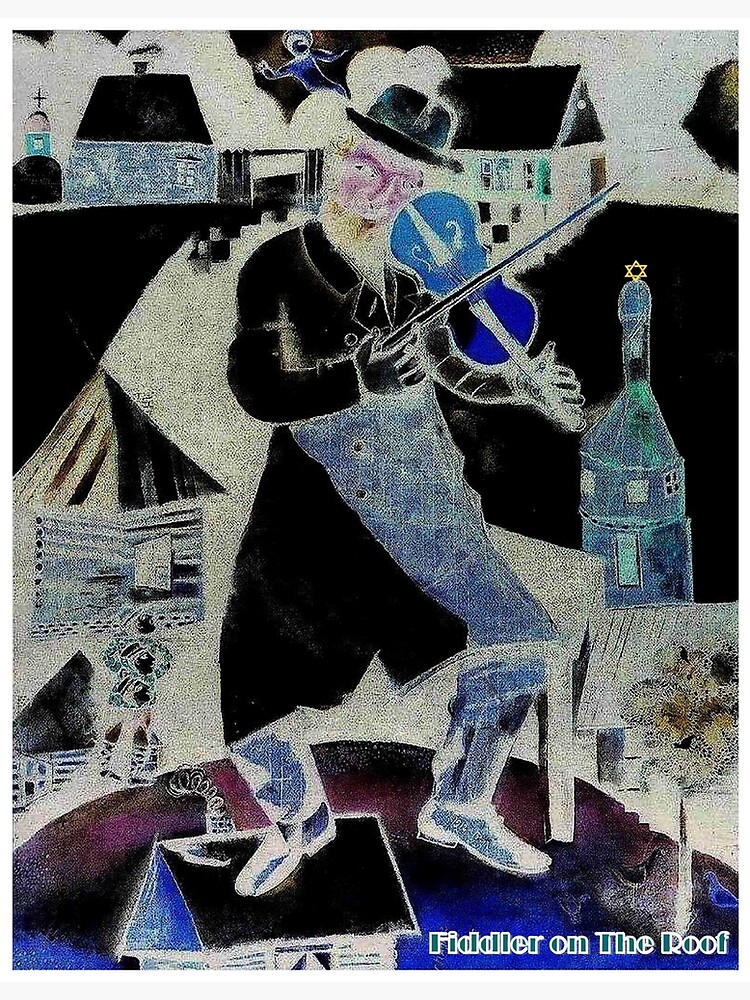This vertical rectangular illustration, an abstract homage to the musical "Fiddler on the Roof," features a central figure of a man playing a blue violin. The man stands at the forefront, characterized by his long black coat, part of which is blue, black boots, and a black bowler hat. His distinctive features include a long white beard and hair. At the bottom right corner of the image, the title "Fiddler on the Roof" is prominently displayed in blue letters with a white outline. Surrounding the fiddler, the background is a blend of various buildings: a hut-like house with a steep roof beneath his feet, and a mix of larger structures above, including one with a dome and cross, possibly a church. Additional buildings, some with chimneys emitting smoke, contribute to the intricate scene, enhanced by a black roadway leading into the composition. The abstract elements combined with detailed depictions of buildings evoke a surreal yet poignant atmosphere reflective of the musical's themes.